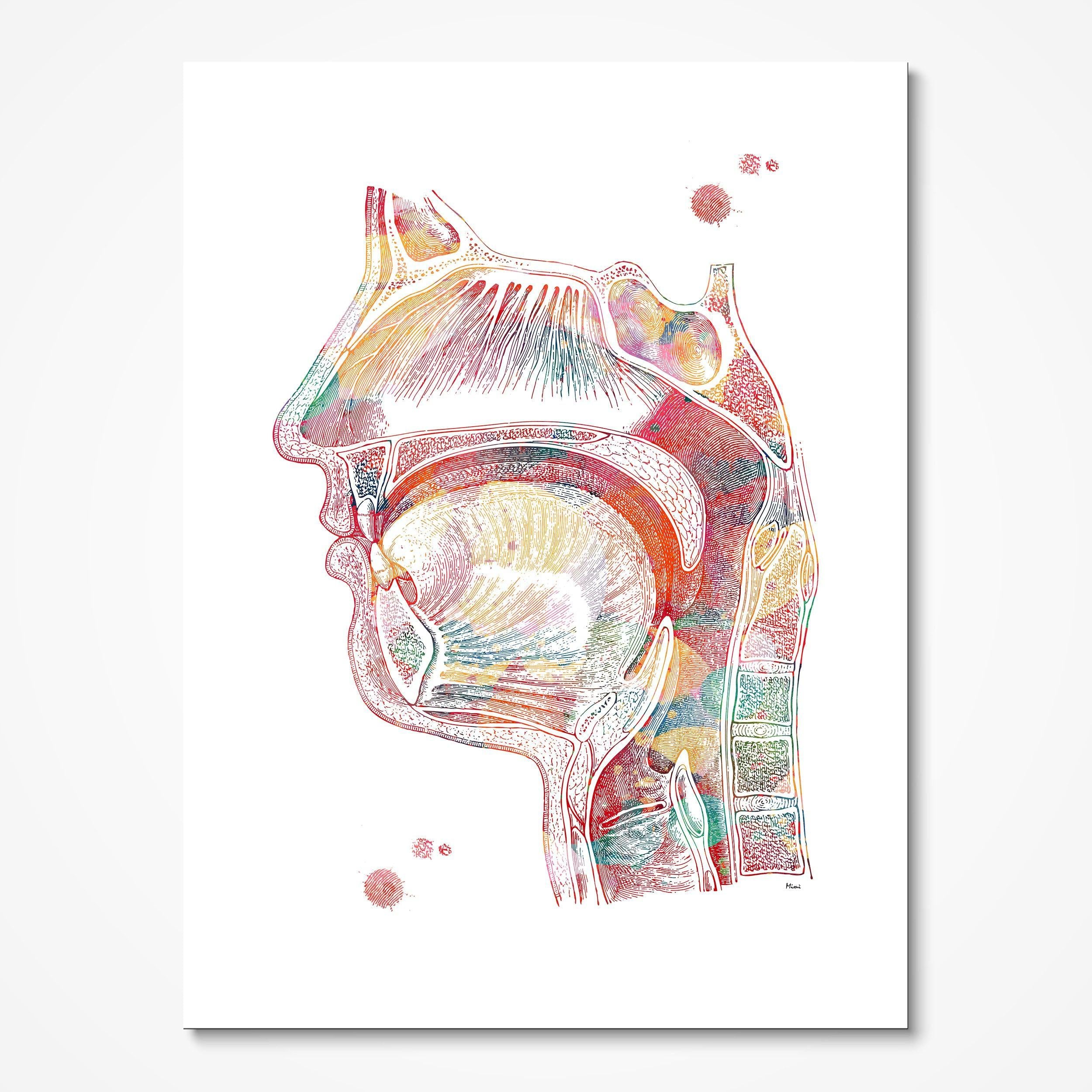The image is a detailed and colorful anatomical drawing displayed on a white background, closely resembling a biology textbook illustration. It features a profile of a human head, highlighting various internal structures such as the muscles, sinuses, esophagus, and spinal cord with vibrant colors including red, yellow, pink, green, and blue to differentiate the parts. The drawing does not have labels, which highlights its artistic nature despite its educational content. The image is centered on the head, nose, mouth, and associated structures, and includes a small black signature in the lower right corner, potentially the artist's initials. It serves as both an anatomical study and a visually engaging educational piece.